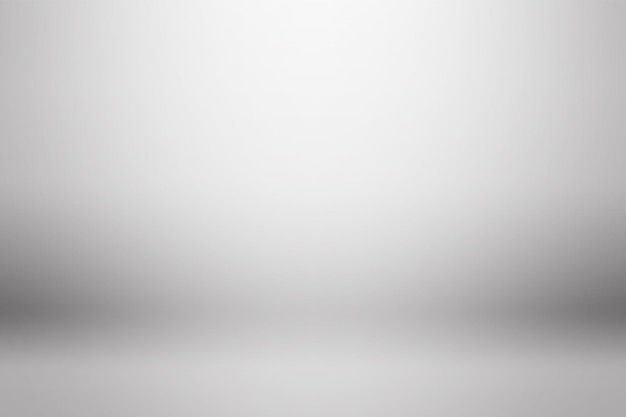The photograph is a horizontal rectangle predominantly displaying a blurry white wall, contributing to its minimalistic nature. There is a gradient effect throughout the image, with the top and center appearing brighter white, gradually shading into light gray towards the edges. Approximately three-quarters down the image, darker black shades emerge on both sides, though the center remains lighter. Some dark spots hint at possible shadows or figures lost to the blur. This gives the impression of viewing the crease of a vertically held, open book. However, the entire image lacks focus, making any specific elements indiscernible.